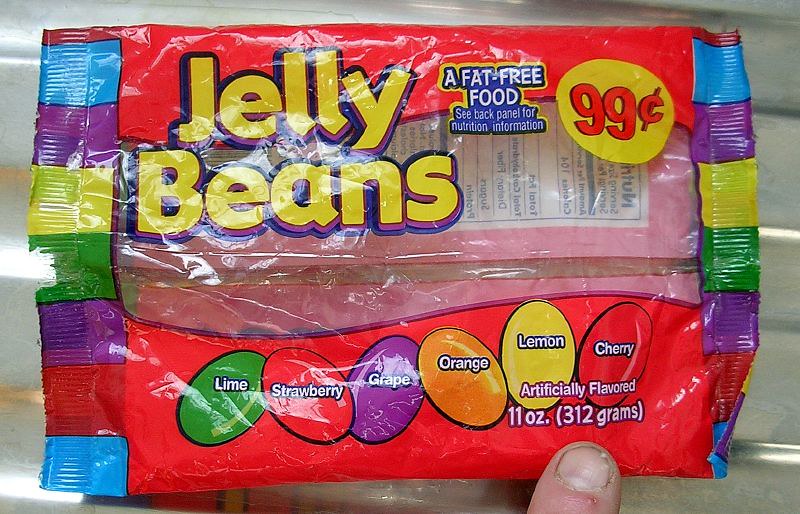An indoor, close-up photograph captures an empty, clear bag of jelly beans, predominantly red at the top and bottom edges. Emphasis is placed on the colorful variety of jelly beans it once contained, including flavors like lime, strawberry, grape, orange, lemon, and cherry, each illustrated on the packaging. The bag prominently features yellow and red text, stating "jelly beans" and "99 cents" within a big yellow dot, and notes that it is a fat-free food. The product's detailed labels also indicate it's artificially flavored, weighing 11 ounces (312 grams). Intriguingly, the edge of the bag is decorated in a rainbow pattern featuring Carolina blue, purple, yellow, green, purple, red, and blue. The image highlights a visibly dirty index finger, possibly from someone who performs manual labor, pointing towards the text. The nail is unkempt, exhibiting dirt and damage, and the finger shows signs of wear, adding a gritty aspect to the photo. The bag is held over a silver, corrugated steel tray, suggesting an industrial or kitchen setting.